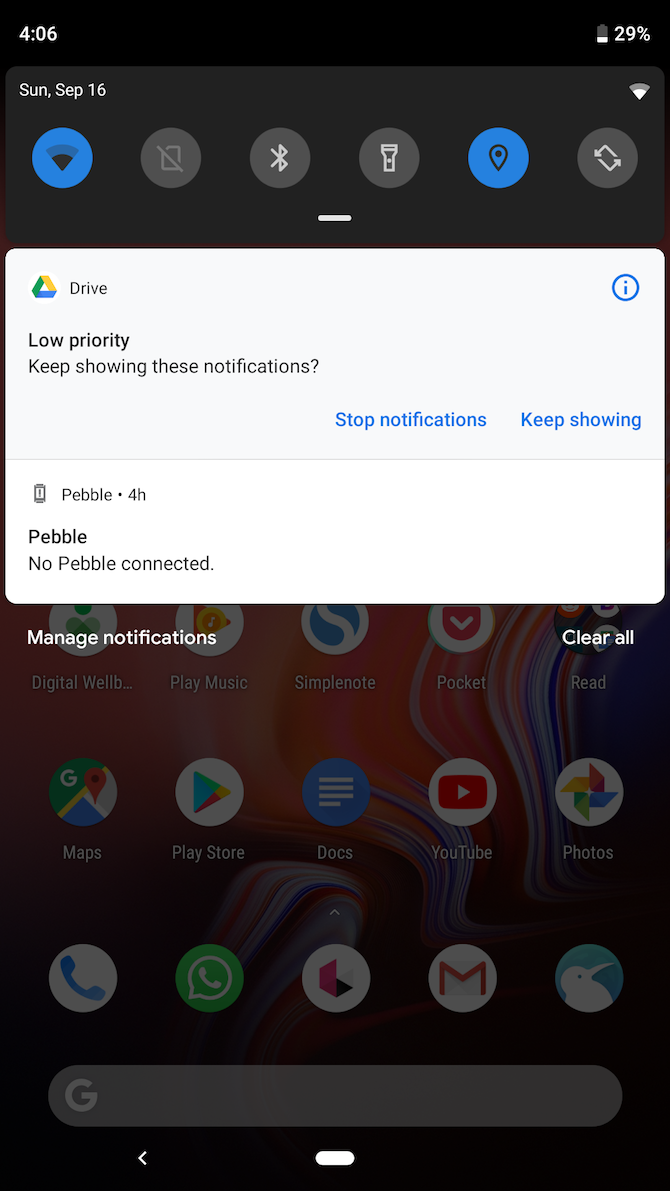Here is a cleaned-up and detailed caption for the image:

---

This screenshot shows the home screen of a smartphone. At the top left corner of the screen, it displays the current time, 4:06, and the battery level at 29%. Below this, there's a gray bar indicating the date as Sunday, September 16th. Beneath the date, there are six icons, with two of them being blue.

A thin white line separates this section from a notification area below. In this notification section, there is a white box with the Google Drive logo on it and the word "Drive" written next to it. Inside the box is a lowercase "i" within a circle. Below the Drive logo, the text reads "Low priority, keep showing these notifications." There are two blue buttons labeled "Stop notification" and "Keep showing."

Further down within the white box, there's a mention of "Pebble" indicating a duration of four hours with a notification stating "No Pebble connected."

Outside the notification box, at the bottom of the screen, there are options to "Manage notification" and "Clear all notifications."

The desktop background of the phone displays several app icons, including those for YouTube and Google Maps. At the bottom, there is a gray Google search bar with a "G" on its left side.